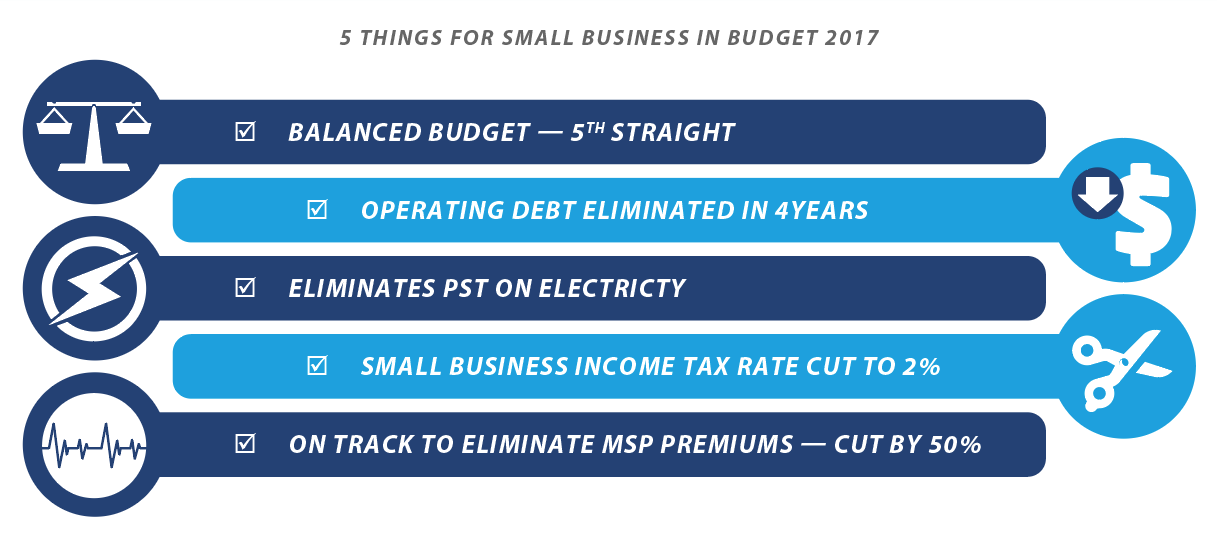This infographic with a white background and varying shades of blue stripes presents five key points from the 2017 budget relevant to small businesses. At the top, a grey header reads, "Five things for small businesses in budget 2017." Each point is detailed within a horizontal section.

1. The first section, with a dark blue stripe and a scale icon in a blue circle on the left, states, "Balanced budget, fifth straight."
2. Following that, a lighter blue stripe with a dollar sign and downward-pointing arrow icon on the right notes, "Operating debt eliminated in four years."
3. Next, a darker blue stripe with a lightning bolt icon on the left declares, "Eliminates PST on electricity."
4. The fourth section in light blue, featuring a scissors icon on the right, announces, "Small business income tax rate cut to 2%."
5. Finally, a dark blue section with a heartbeat symbol icon on the left reads, "On track to eliminate MSP premiums cut by 50%."

Each icon punctuates the importance of these budgetary measures, making the infographic both informative and visually engaging.